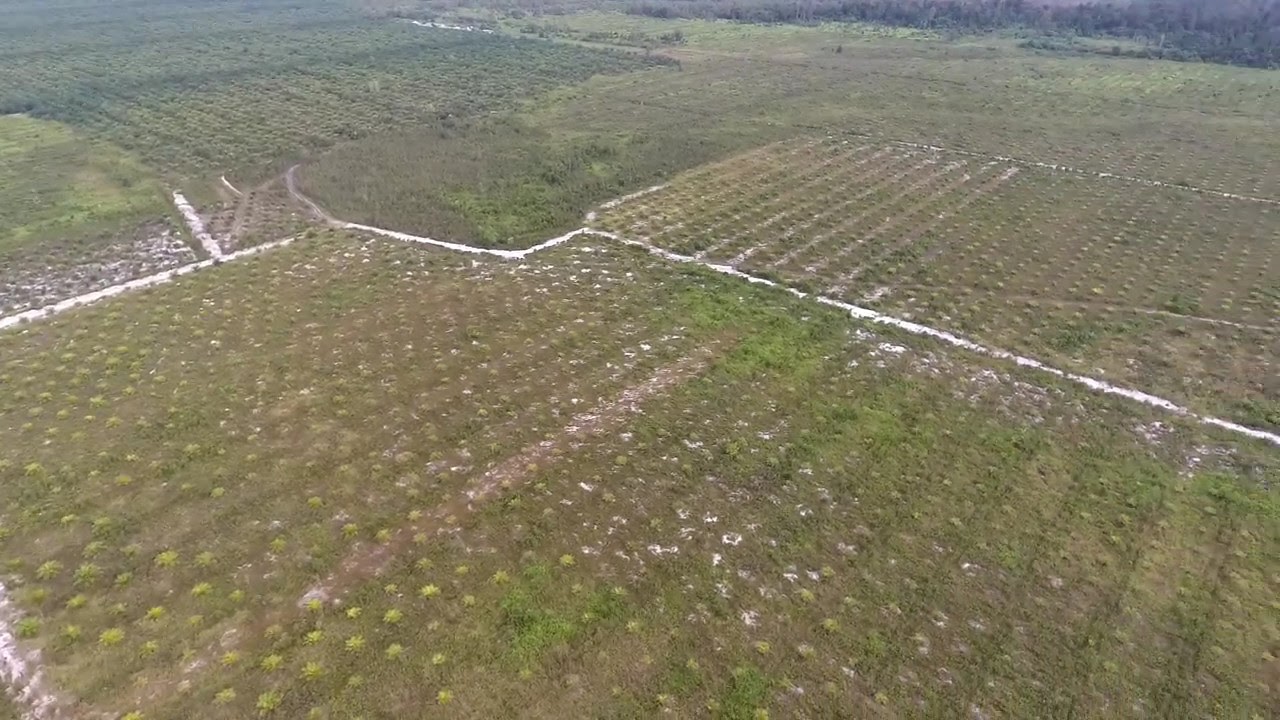This aerial photograph showcases an expansive countryside featuring a patchwork of interconnected farms with varying shades of green and brown. The landscape is segmented into numerous plots, including large and small rectangles and squares. Predominantly light green with patches of darker green and brown hues, the fields display rows of crops interspersed with occasional weeds that create a textured appearance. White PVC irrigation pipes create a zigzag pattern, starting from the center right, moving upward, then veering back down toward the left before continuing to the edge of the image. Notably, there are white specks scattered across the ground, possibly remnants of harvested crops or other material. In the upper left quadrant, vegetation appears denser and taller compared to the other sections. Near the center of the image, a small grove of brush interrupts the uniformity of the crops. Additionally, a line of grayish brush is visible in the background at the top of the photograph, adding depth to the scene.